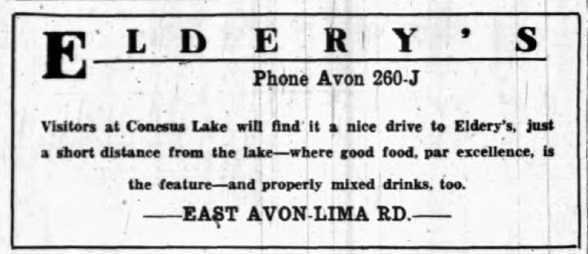The image features an old-fashioned advertisement for a restaurant named "Elderies," positioned horizontally. The ad is designed on a piece of paper with a white background and black text, bordered by a horizontal black line. The text reads: "Elderies, phone Avon 260 J. Visitors at Kinesis Lake will find it a nice drive to Elderies, just a short distance from the lake, where good food par excellence is the feature and properly mixed drinks." Below this, in all capital letters, it states "East Avon Lima RD." The image appears to be a flawed copy with noticeable vertical streaks, likely resulting from smeared ink during the printing process. The ad aims to attract tourists by highlighting the restaurant's proximity to Kinesis Lake and promising excellent food and drinks.